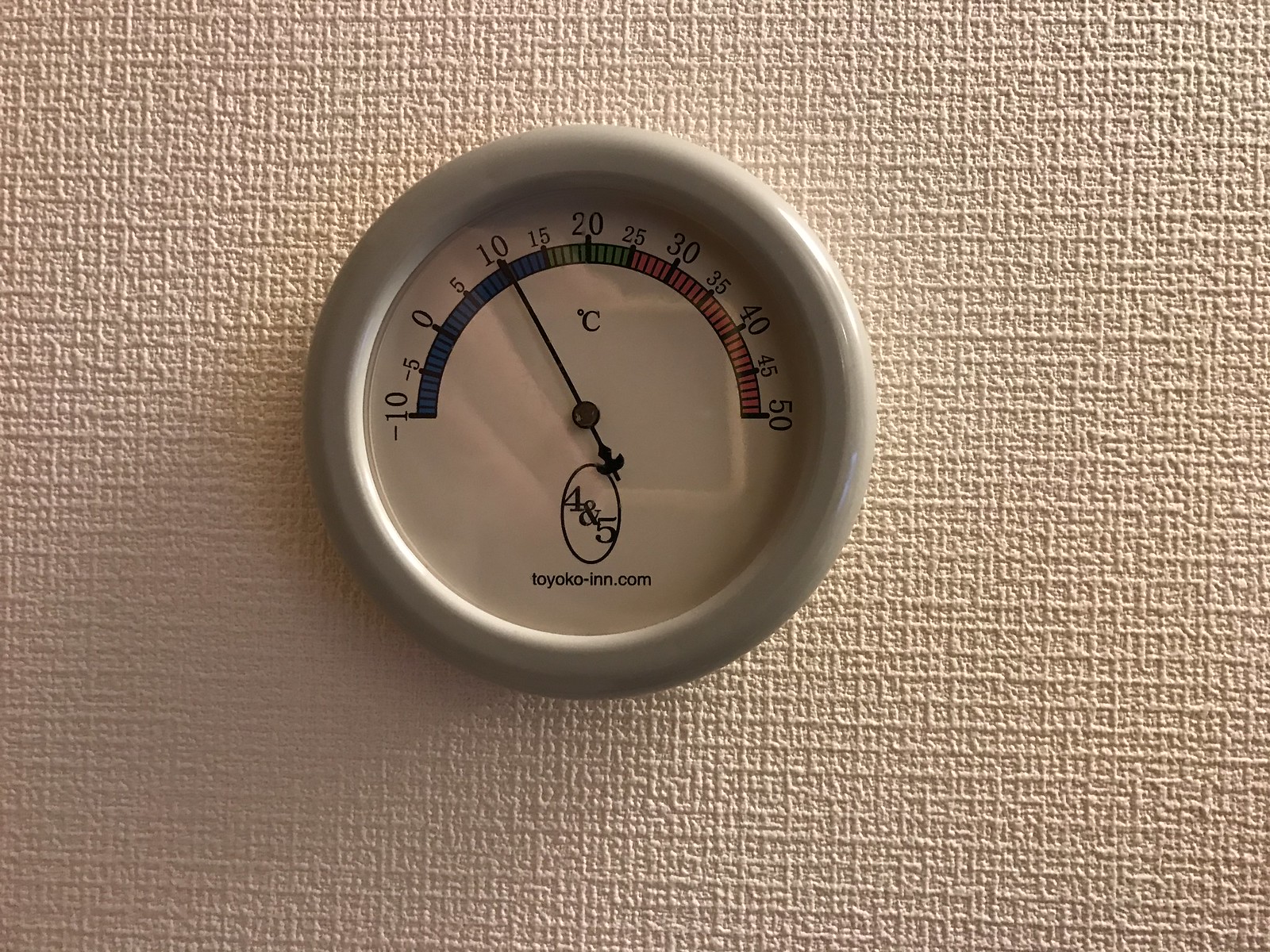The image is a color photograph in landscape orientation, showcasing a mechanical analogue thermometer mounted on a heavily textured wall. The wall appears to be covered with wallpaper featuring a three-dimensional, undulating grid-like pattern of vertical and horizontal lines, almost forming a mesh. The texture is tactile, and the wall's color is a very light orangey-pink.

The thermometer itself is round with a thick, light grey bezel enclosing it. A light source from the top right casts a slight white reflection on the bezel at approximately the two o'clock position. The thermometer is covered with a transparent glass or plastic, reflecting the photographer's hand holding a phone in landscape orientation, which has a yellow case or bezel.

The thermometer's dial spans from -10 to 50 degrees Celsius, displayed in an arch across the top. Below the arch, a degrees Celsius symbol indicates the units of measurement. The color gradient of the dial transitions from black at the -10 mark, through shades of green between -15 and 25, and into shades of orange to red approaching the 50 degree mark. A single black needle points to the current temperature of 10 degrees Celsius.

The brand name, "toyoko-inn.com" (with two 'n's), is prominently stamped on the thermometer. Additionally, there is a vertical oval with a black outline displaying the numbers "4 & 5" diagonally from the top left to the bottom right.